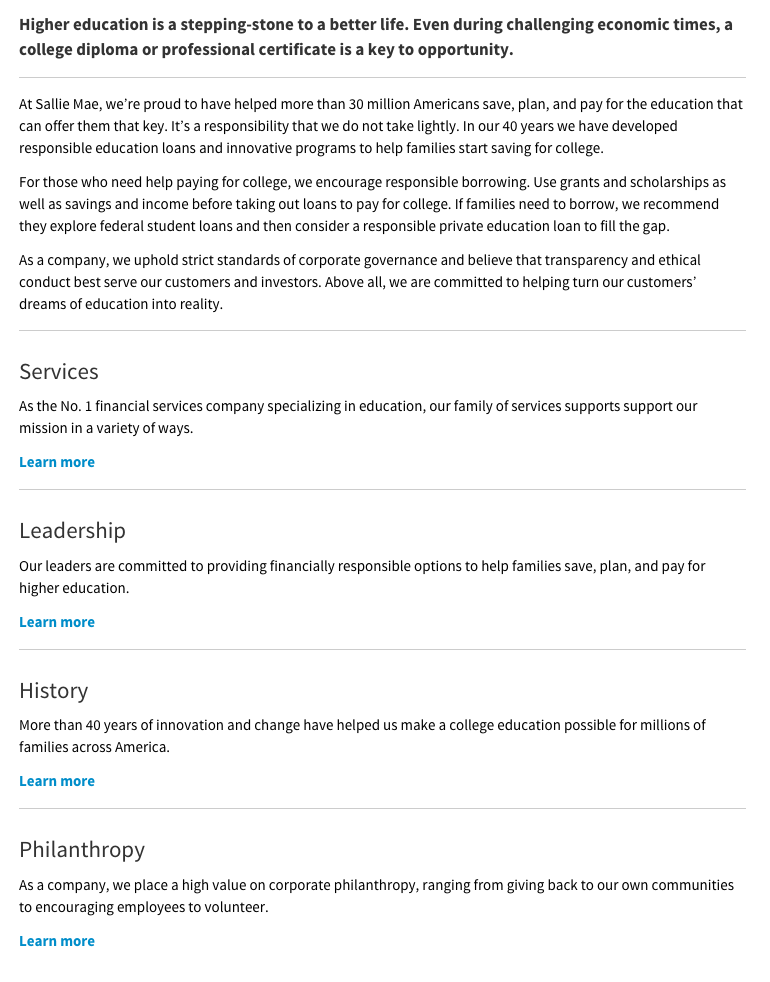Screenshot of a website with a focus on education and financial planning. The page is text-heavy with no images. At the very top, a prominent heading reads: "Higher education is a stepping stone to a better life even during challenging economic times. A college diploma or professional certificate is a key to opportunity." Below this, the website states that Sallie Mae is proud to have assisted over 30 million Americans in saving, planning, and paying for their education over the past 40 years. The company emphasizes its commitment to responsible education loans and innovative savings programs aimed at helping families prepare for college expenses. It advises utilizing grants, scholarships, savings, and income before taking out loans for college. If borrowing is necessary, Sallie Mae recommends exploring federal student loans first and then considering responsible private education loans to cover any remaining costs.

The website also underscores Sallie Mae's adherence to strict corporate governance standards, transparency, and ethical conduct to best serve their customers and investors. A clear commitment is expressed to help customers achieve their educational dreams.

Four main sections are highlighted: "Service," "Leadership," "History," and "Philanthropy," each containing brief descriptions pertaining to these topics. The comprehensive and detailed text outlines the company's mission, values, and services aimed at supporting educational aspirations.